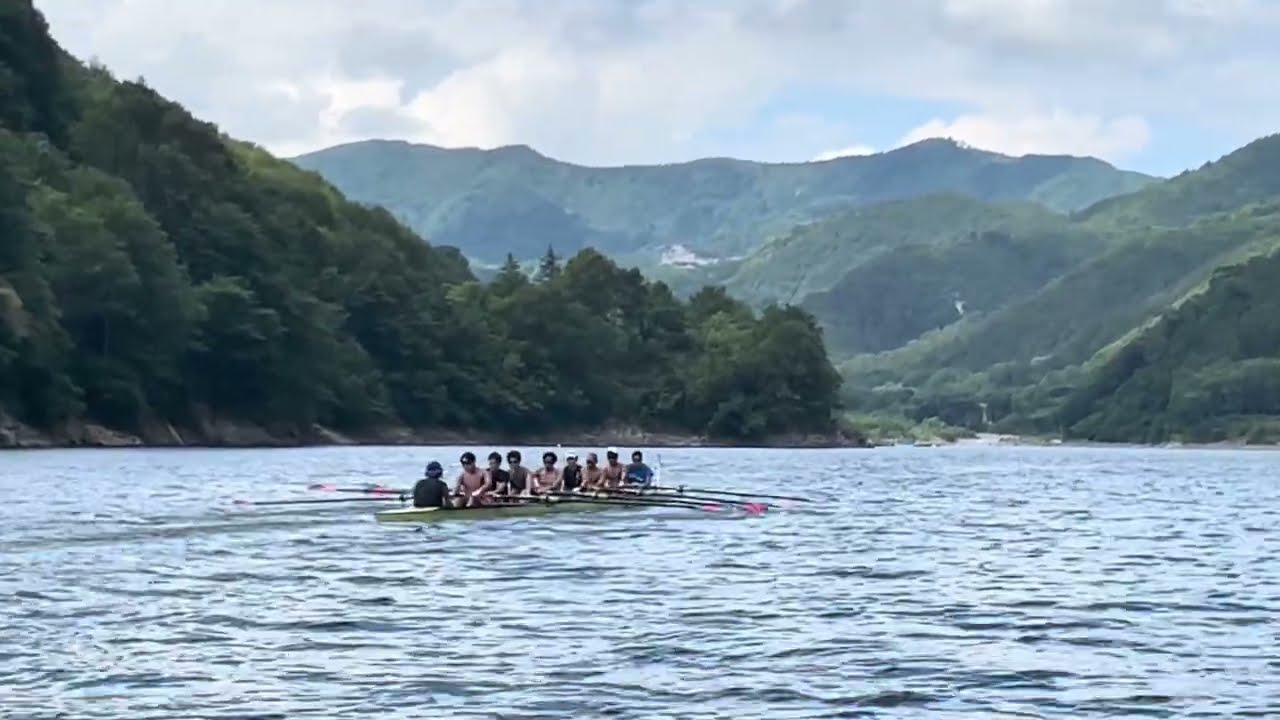The image depicts a long, narrow, yellow rowboat situated in the calm, blue waters of a large lake. There are nine men seated in the boat, with one man at the front, wearing a black shirt and facing the others, who are seated in a line and holding black oars extending into the water. The scene is set in a tranquil, rural area with no other boats or people around. The backdrop features a range of hills and mountains, covered in lush, green trees, with some rocky patches visible towards the shoreline. In the distance, the hills form a continuous outline from left to right, with a valley or river opening at the center-right of the image. The sky above is mostly clouded, with patches of blue peeking through, adding to the serene and picturesque atmosphere.